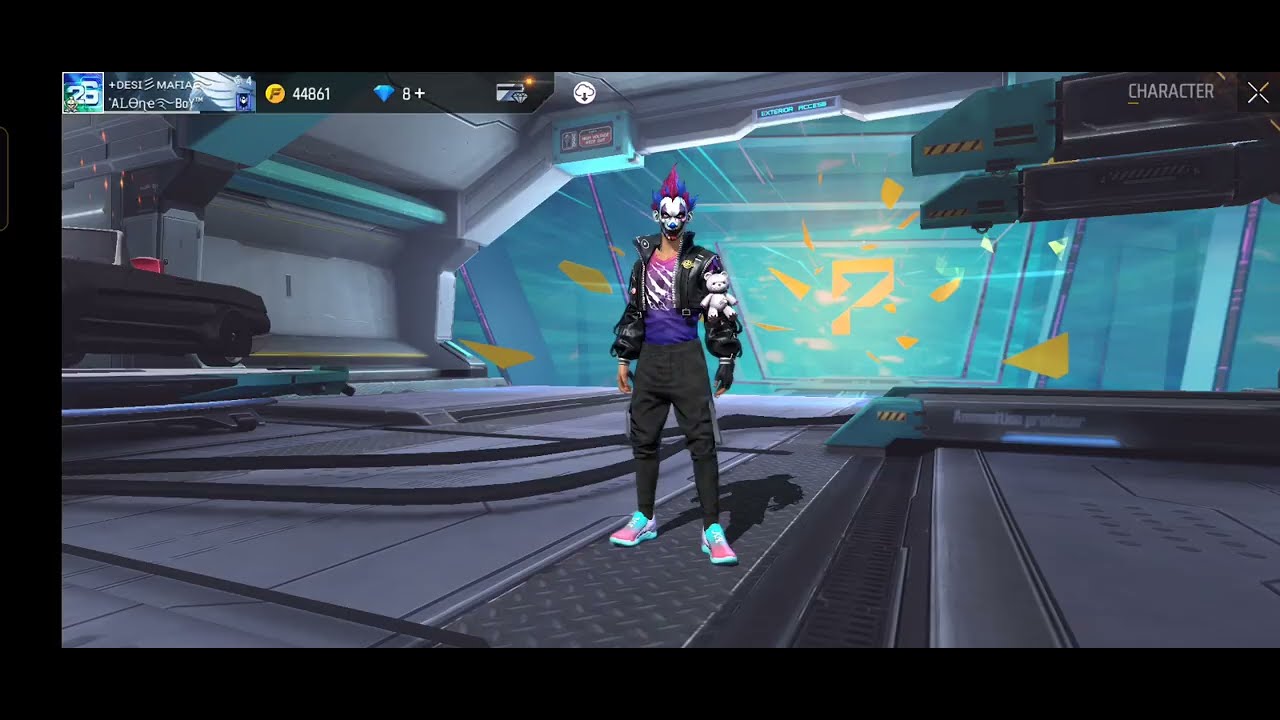This screenshot from a video game features the main character prominently standing in what resembles a spaceship corridor with a hammered metal floor and a turquoise background accented by yellow blotches. The character gives off a punk-rock vibe, portrayed as a sinister punk clown with spiky purple and pink mohawk hair. His face is painted white with a menacing black smile and exaggerated eyebrows. He sports a short, cropped leather jacket with fluffy sleeves, to which a white teddy bear is attached. His attire includes black pants adorned with gray straps and pastel pink, blue, and turquoise ombre sneakers. The character also wears an ombre shirt transitioning from pink to purple with some white lines. 

In the user interface, the top right-hand corner displays the word "character" followed by an 'X'. On the top left, there is a banner featuring the number 26 inside a square, an unreadable name, a golden coin labeled "44861," a diamond marked with "8+," and additional icons including what seems to be a credit card and another diamond. This detailed visage of a punk clown in a technologically futuristic backdrop combines elements of whimsy and menace, creating a striking visual impact in the game's character selection or lobby screen.